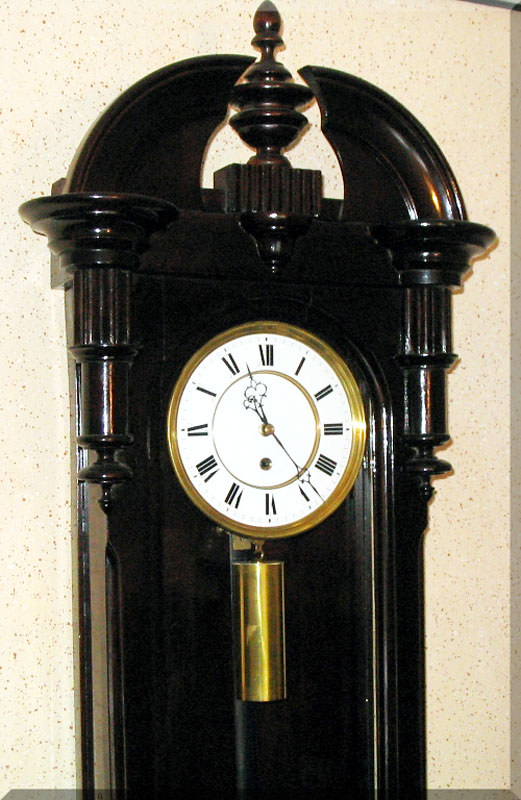The photo captures an old grandfather clock standing against an off-white, speckled wallpaper, evoking a vintage 1960s or 1970s aesthetic. The clock, in excellent condition, is crafted from a dark brown, nearly black, lacquered wood. Its relatively small clock face is enclosed within this black wooden structure, featuring a distinctive gold outer rim and Roman numerals for time markers. The clock displays an hour and a minute hand, with no second hand visible, indicating the time around 11:20. Below the clock face, a large gold pendulum is prominently displayed behind the glass casing. At the top of the structure, there are two arches that lead to a pointed detail, reinforcing its classic design.